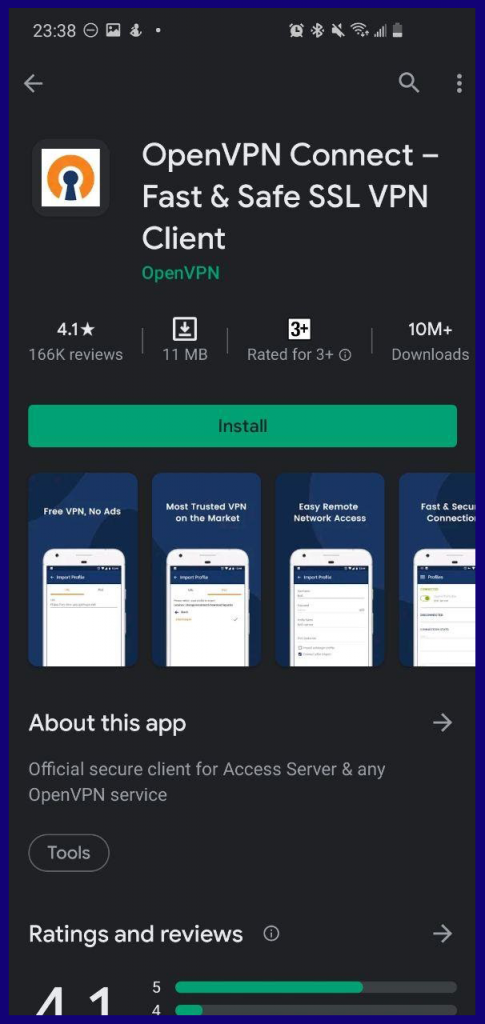The image is a vertical screenshot captured on a smartphone, evidenced by the layout and various status indicators. The time displayed is 23:38 or 11:38 p.m. The user has 'Do Not Disturb' mode activated, and the screenshot was just taken. Several icons are visible, indicating that there is an active alarm, Bluetooth is connected, the phone is muted, Wi-Fi is connected, and the reception and battery levels are displayed.

The screenshot depicts a page from the Google Play Store, featuring an app called "OpenVPN Connect - Fast & Safe SSL VPN Client." The app's name is in white font, while the developer's name, OpenVPN, is shown in green font, suggesting it is clickable to view other apps by the same developer. To the left of the app name is the app's icon.

Beneath the app name, various user reviews and ratings are visible. The app has an average rating of 4.1 stars based on 166,000 reviews. It requires 11 megabytes of storage space and is rated suitable for users aged three years and older. The app has been downloaded 10 million times.

A green box with black font displays an "Install" button. Below the installation section, several images showcase the app's features and user interface. Further down, in white font, there is an option to select "About this app," which provides a brief description and additional details, including the app's category and more extensive information about its ratings and reviews.